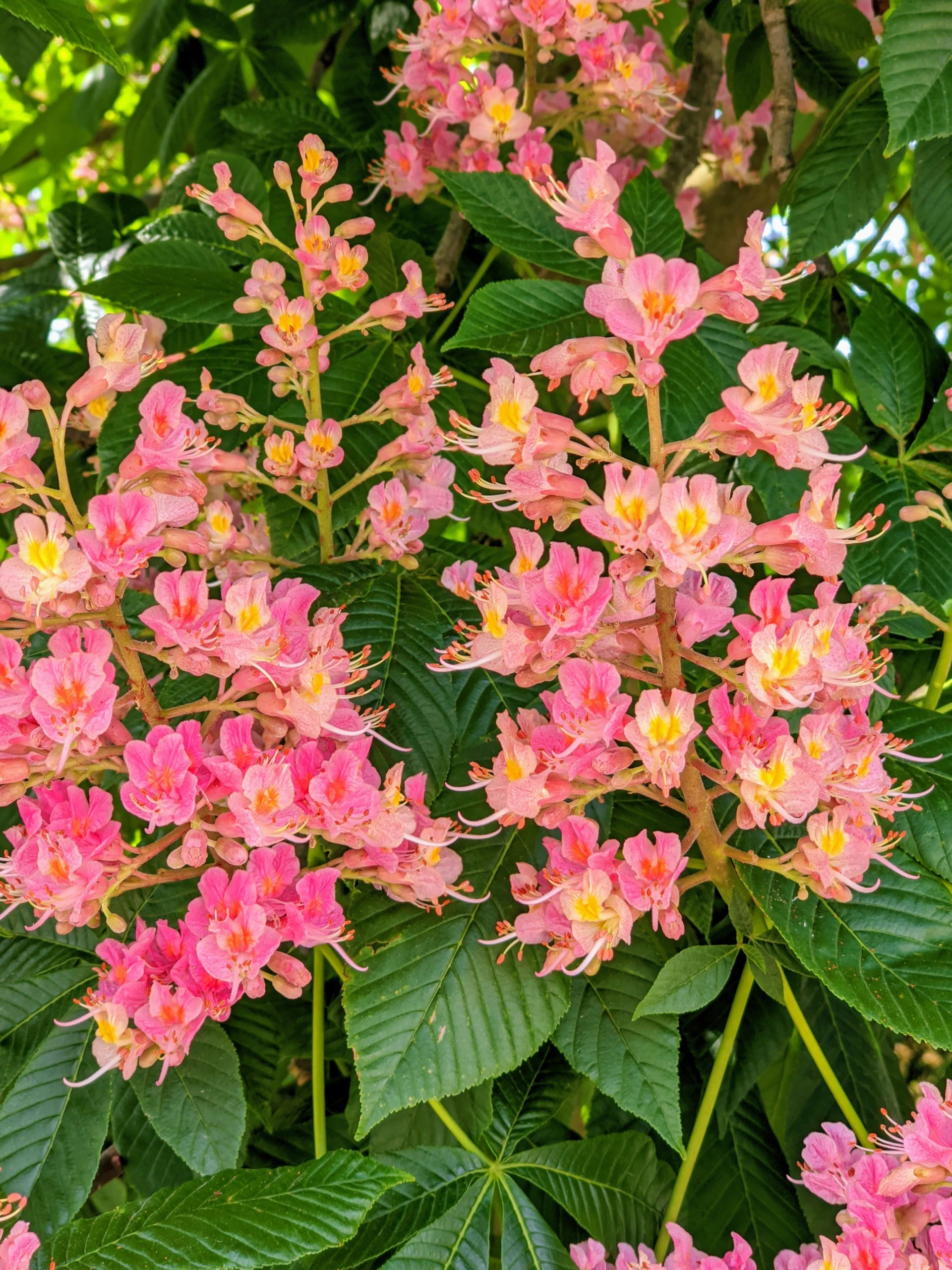This photograph captures a vibrant cluster of bright pink flowers with yellow centers, possibly resembling snapdragons or orchids. The flowers, which range from darker pink to lighter pink, bloom profusely in clusters, each flower showcasing four to five delicate petals. A prominent pink floral structure extends from the center of the petals, adding to the intricate beauty of the blossoms. These eye-catching blooms are set against a lush backdrop of large, wide, green leaves with pronounced lines and intricate veining, evoking a tropical ambiance. The entire background is filled with foliage, with dappled sunlight filtering through the leaves, creating a play of light and shadow that enhances the overall vivid and tropical feel of the scene.